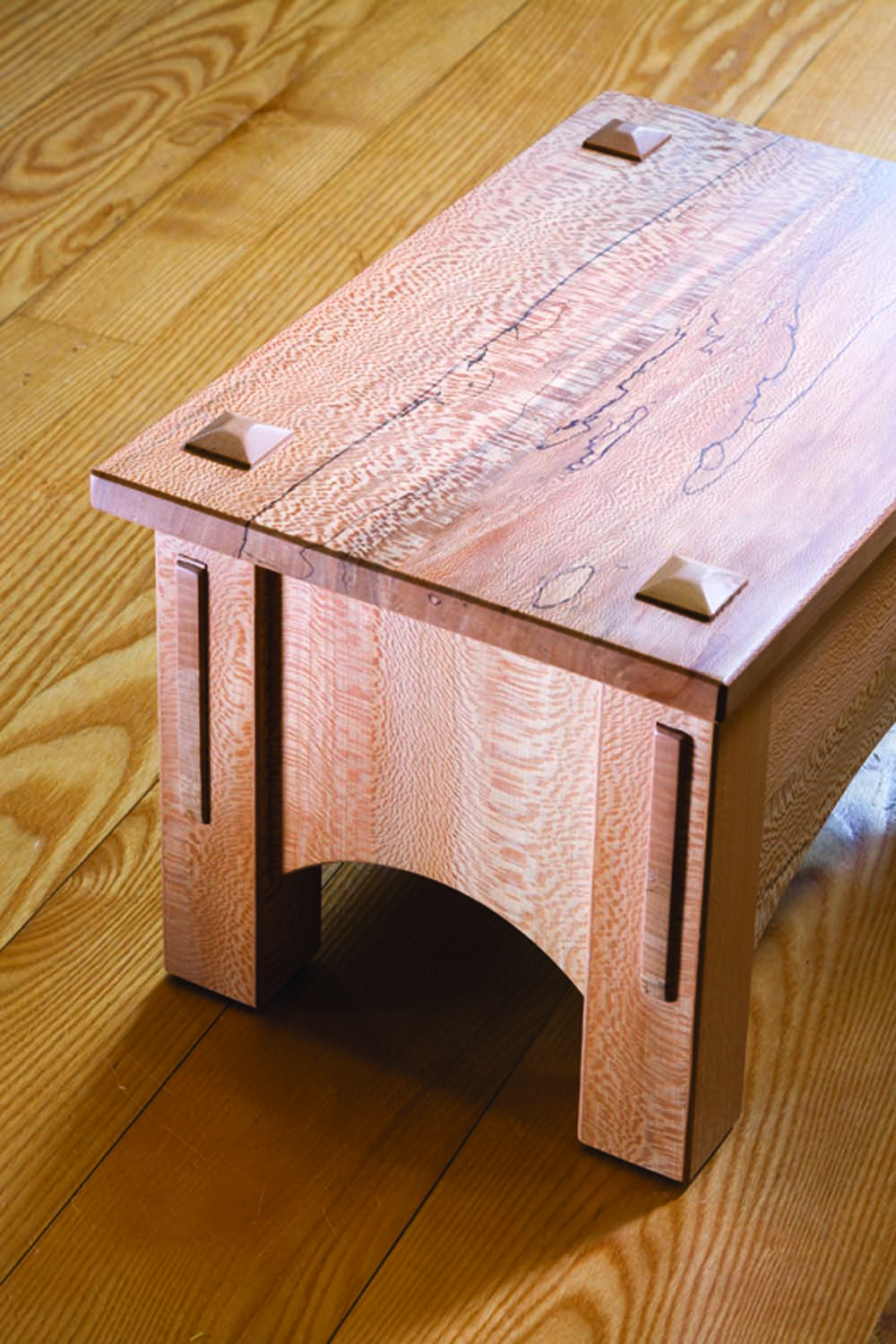The photograph features a small, handmade wooden step stool placed on a light brown, hardwood floor composed of various finished planks. The stool's craftsmanship is evident; it has a smooth top and four legs, with a shadow beneath it suggesting back legs are present. Each corner of the stool's top has a raised square, though the photograph is angled such that one corner is obscured. An arch can be seen on the short end of the stool, adding to its decorative appearance. The setting appears to be a sunny room, captured close up with no other objects in view, showcasing the floor’s grains and finish. This stool seems practical for use in spaces like a kitchen or bathroom, possibly for a child to reach higher surfaces.